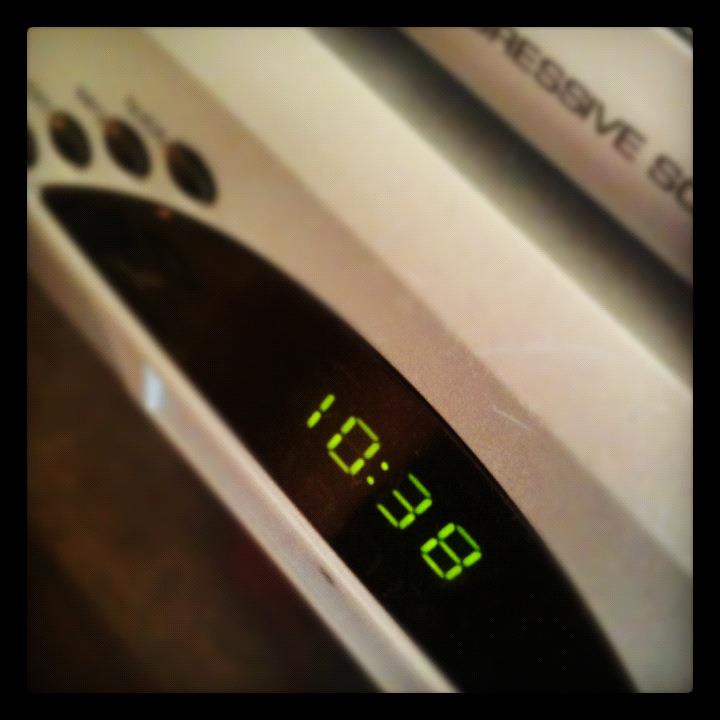This close-up photograph captures the digital clock display of a kitchen appliance, likely a stove, given the surrounding white metal casing. The clock face itself is designed as a semicircle with a flat bottom and rounded top. The numbers, displayed in a green, calculator-like text, indicate the time as 10:38. Along the right side of the clock face are four buttons arranged vertically. In the upper right-hand corner of the image, partial black text is visible with the letters "RESSIVE" and an isolated "S," suggesting that the full word might be "PROGRESSIVE" before being truncated.